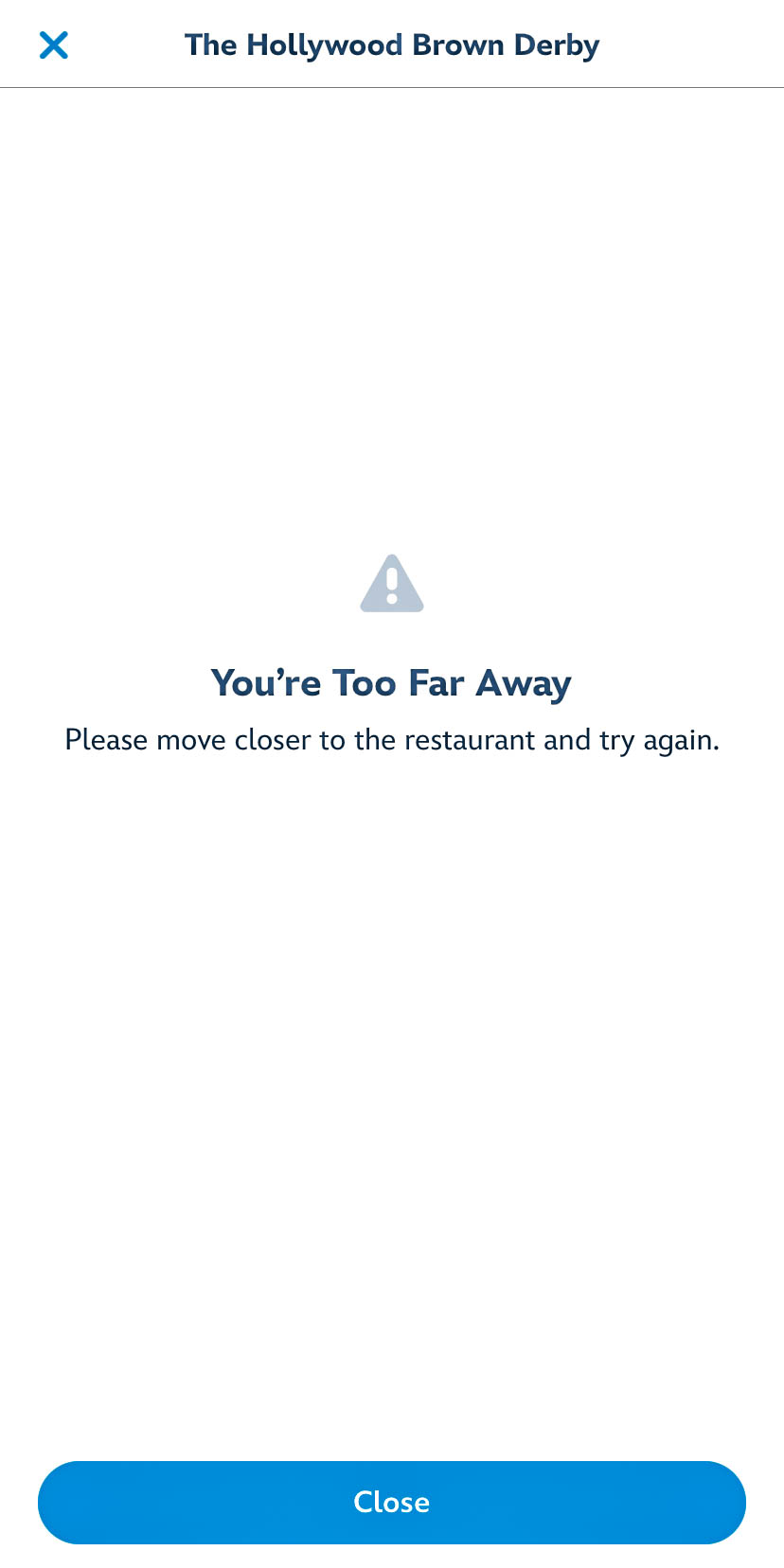The image features a predominantly white background. In the top left corner, there is a blue "X" symbol. Centered at the top in black text are the words "The Hollywood Brown Derby." Beneath this title, a light gray line extends horizontally from left to right. 

Taking up the middle of the image, there is a gray triangle with an exclamation mark inside it, signaling a warning or alert. Below this triangle, bold black text reads, "You're too far away." In smaller, non-bold text underneath, the message continues, "Please move closer to the restaurant and try again."

The lower section of the image contains a significant amount of empty space, culminating at the very bottom with an oblong, dark blue button. The button features the word "Close" in white letters.

Overall, the image is marked by ample white space, with minimal additional elements or details.